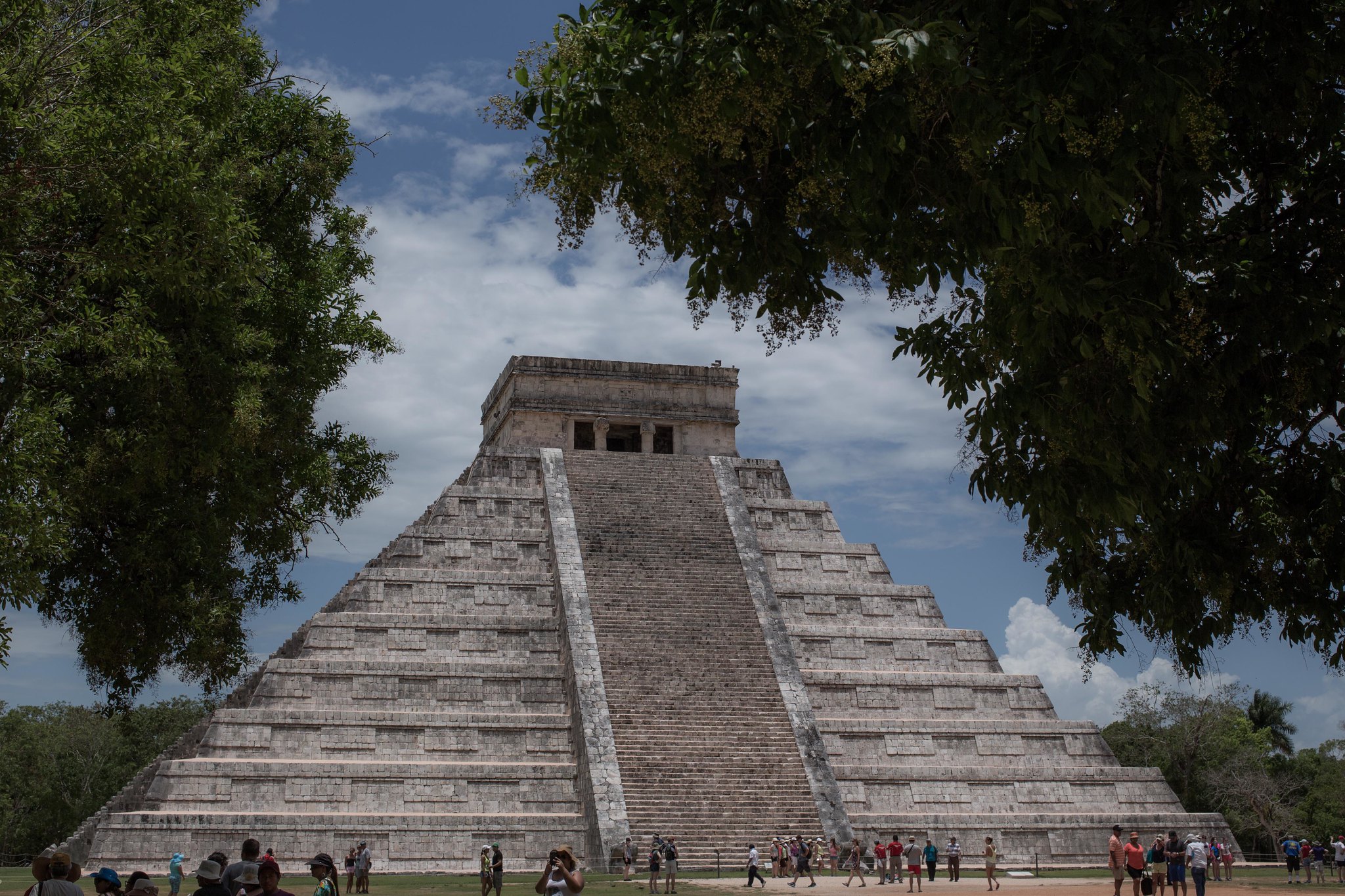The photograph captures an impressive ancient stone structure, likely a South American temple or shrine, characterized by its tiered design with multiple flat levels. Unlike traditional pyramids, this structure has a flat top, more reminiscent of a temple. Prominent stone stairs ascend the sides, suggesting accessibility to the upper levels, although no people are visible at the top—possibly restricted for safety reasons. At the base, several tourists are gathered, providing a sense of scale to the monument. The scene is framed by lush, large trees and set against a partly cloudy blue sky on what appears to be a sunny day. The image has no accompanying text.